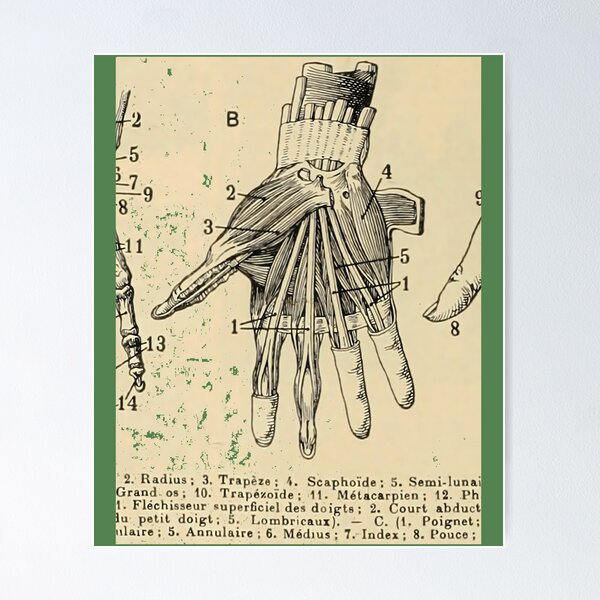This is a detailed vintage anatomical drawing of a human right hand, depicting the muscles and tendons with the skin meticulously peeled back to reveal the underlying structures. The main hand, oriented with the palm facing the viewer, is surrounded by various numbers that pinpoint specific anatomical features. Accompanying these numbers, a comprehensive key at the bottom of the image lists the corresponding muscles and tendons, although some terminology appears to be in French, including terms like "radius," "trapeze," "scaphoid," and "semi-lunar grandos." On the left side of the drawing, there's a partially visible representation of another hand, focusing on the skeletal bones, while on the right, a normal finger with a nail points towards the central hand. The diagram seems to be part of an old anatomy textbook and is set against a plain white background, highlighting the intricate details of the hand's anatomy.